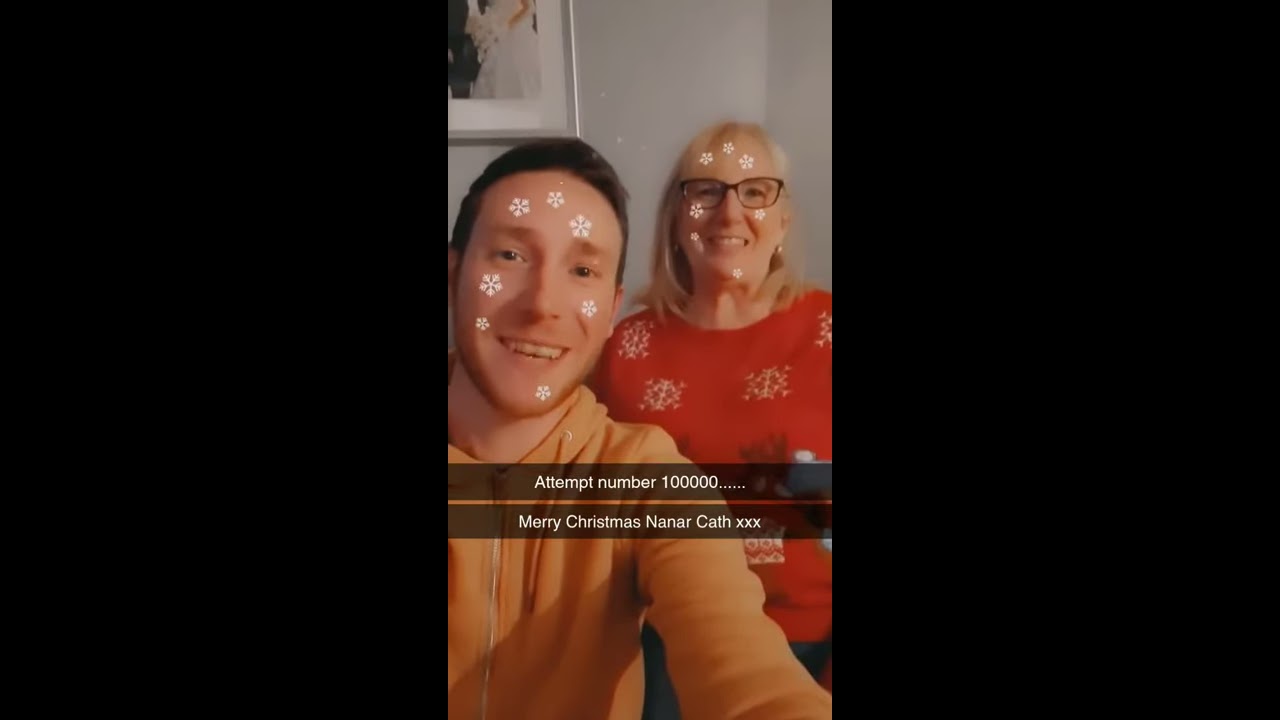In this indoor holiday-themed photograph, an older woman with blonde hair, black glasses, and a red sweater adorned with snowflakes stands partially behind a younger man with black hair and stubble, dressed in a yellow or orange hoodie. The image features a festive snowflake filter overlaying both their faces, adding a wintry touch. Despite the Christmas greeting, which reads "Merry Christmas Nayanar Cam" followed by "attempt number 100,000," the setting lacks overt Christmas decorations. A partial view of a painting in a silver frame is visible on the plain wall behind them, contributing subtly to the room's ambiance. The photograph, likely a screenshot from an Instagram story or Snapchat, captures a lighthearted holiday moment between the two individuals.